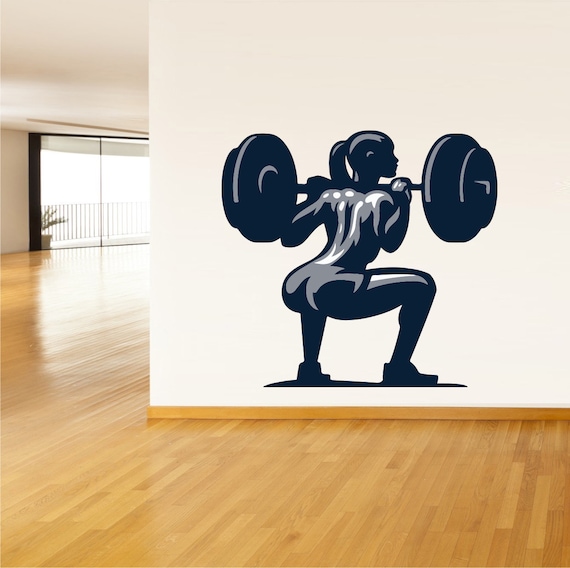A topless woman is captured in mid-squat position, holding a barbell across her shoulders. The barbell features round weights on either end, resting securely on the back of her shoulders. Her athletic build is emphasized by the defined muscles in her buttocks, which are partially visible above her shorts. She is wearing athletic shorts and shoes that accentuate her well-defined calf muscles. The setting is a room with white walls, adorned at the base with brown trim, and the floor consists of shiny brown wooden slats. The white ceiling contrasts with the earthy tones below. To the left side of the frame, there is a sliding glass door, next to which stands a leafy green plant. Outside the door, a metal handrail is partially visible, hinting at an exterior space beyond the room.